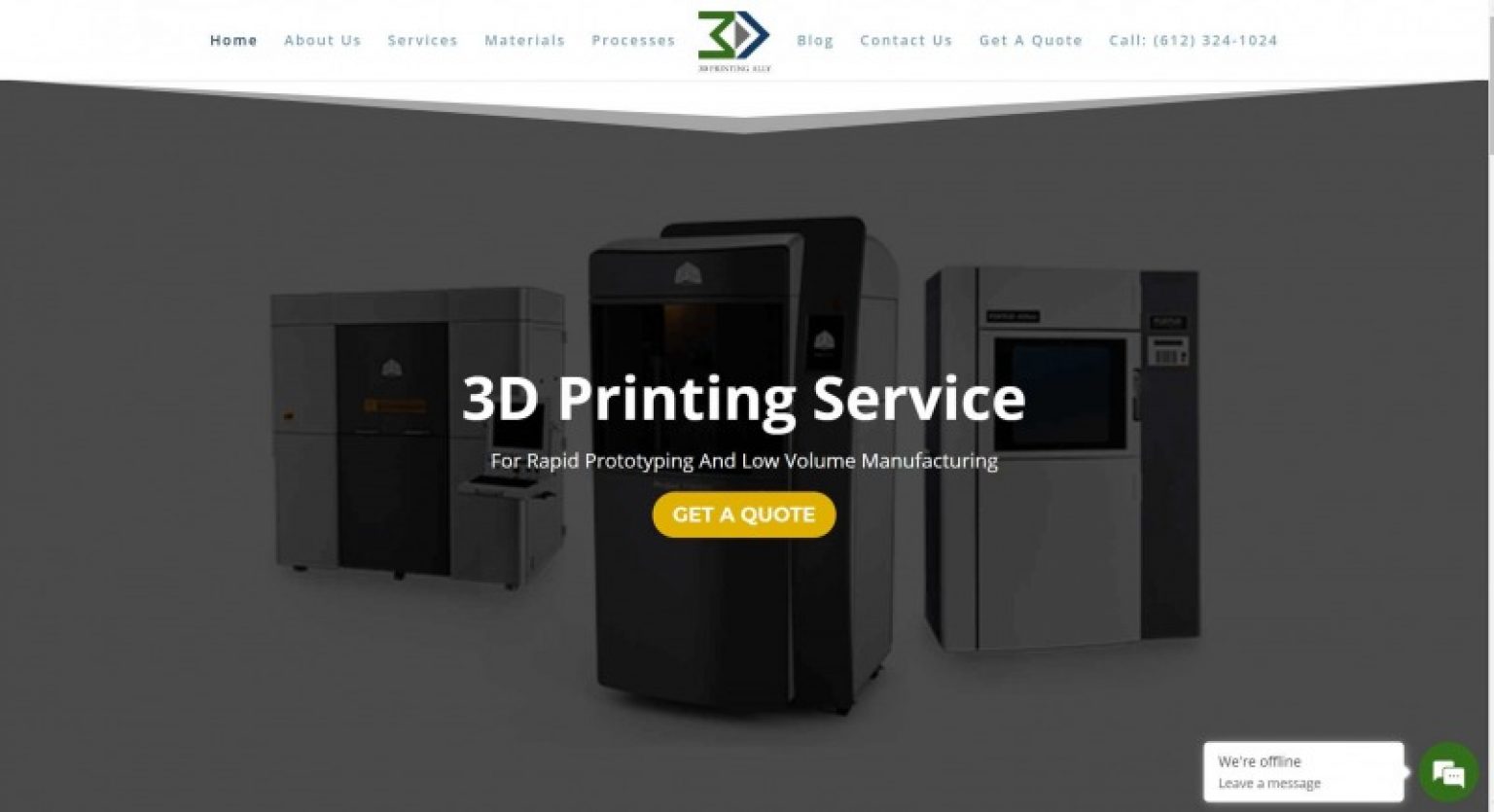The image showcases a 3D printing service interface, with a focus on the company’s logo and navigation menu. The logo, centrally positioned at the top, features a distinctive “3D” design—where the “3” is green and the “D” has a unique pointed accentuation to the right. The navigation menu unfolds as follows: Home, About Us, Services, Materials, Processes. Further to the right of the logo, the options include Blog, Contact Us, Get a Quote, concluding with a “Call” section alongside the phone number 612-324-1024.

Beneath this header, the main picture prominently displays three large 3D printers, indicative of robust industrial capacity. In front of these machines, the words "3D Printing Service" are clearly visible. An inviting "Get Quote" button is also present, encouraging potential customers to make inquiries or request estimates.